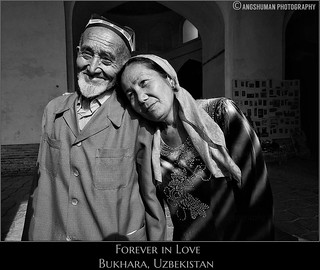This black and white professional photograph, titled "Forever in Love, Bukhara, Uzbekistan," captures an intimate moment between an older couple standing outdoors. The man, who appears to be in his 70s, has a white beard and is wearing a skullcap and a light button-down jacket with pockets on either side. He stands on the left, facing the camera with a gentle smile. To his right, leaning her head on his shoulder, is a woman wearing a kerchief over her head that falls down over her shoulders in the front. She is adorned in a black and white top with a decorative design featuring beads. They are standing on a sidewalk, with the backdrop including a building with a brick bottom and an archway, as well as white and gray painted walls and an iron grill. The upper right of the image is marked "Copyright, Agershman Photography,” indicating that it is a professionally taken picture.